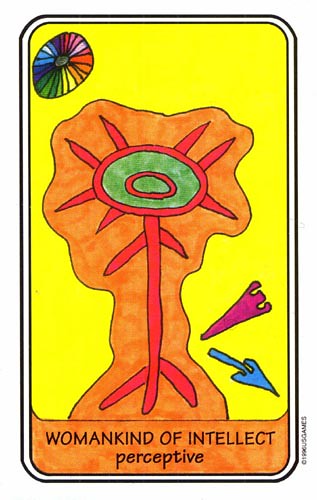This image appears to be the decorative side of a card, possibly a tarot card. It features two black borders with rounded corners; the outer border is slightly thicker than the inner one. Sandwiched between these borders is a white band.

The main section of the card, taking up the top 90%, is a rectangular space with rounded corners and a yellow background. In the upper left corner of this space, there is an abstract, multicolored image that appears to resemble a flower, although it could be interpreted as another imaginative design. The "flower" includes a rich blend of colors: yellow, orange, red, violet, tan, purple, blue, light blue, and various shades of green.

At the focal point of the image, there is a distinctive red stem with red, spike-like protrusions. This connects to a horizontally oriented, red-outlined oval with a green interior and a smaller red oval outline inside it, which houses an even smaller green center. Surrounding these central elements are various irregularly shaped triangles, some resembling arrows, and others appearing as triangles with notched edges. The overall outline of the "flower" is drawn in a dirt-like color, adding a rough, handmade quality to the image.

At the bottom of the card, a bold header reads "WOMANKIND OF INTELLECT" in all capital black letters. Below this, in black lowercase letters, is the word "perceptive".